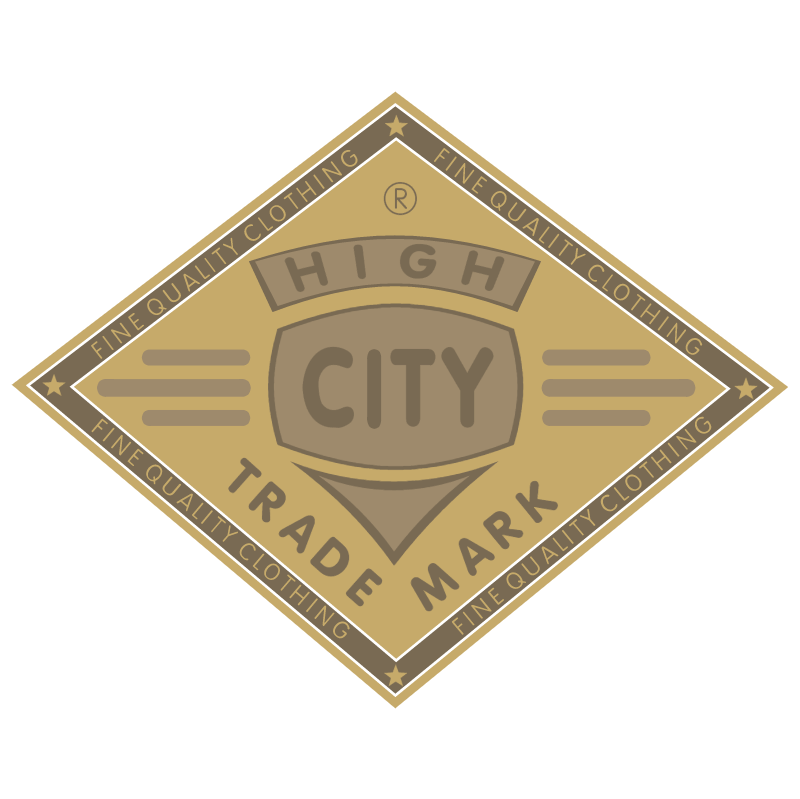The image showcases a diamond-shaped emblem representing a trademark on a plain white background. The emblem features a dark border with a series of color layers: a mustard yellow outer edge, a thin white strip, followed by a thicker dark gray band, another thin white strip, and a mustard yellow center. The dark gray band contains capitalized text, "FINE QUALITY CLOTHING," written on all four sides with a star in each corner. In the mustard center, at the top, there is a "®" symbol indicating a registered trademark. Below this, the word "HI" is written in dark gray within a curved rectangle, and beneath that, the word "CITY" appears in a larger font inside a similarly styled curved rectangle. Flanking "CITY" on both sides are three lines extending outward, and below lies a small triangle. Additionally, on the left inner wall of the diamond-shaped inner structure, the word "TRADE" is inscribed in dark gray, while on the right, the word "MARK" is inscribed, completing the detailed emblem for "HIGH CITY" fine quality clothing trademark.